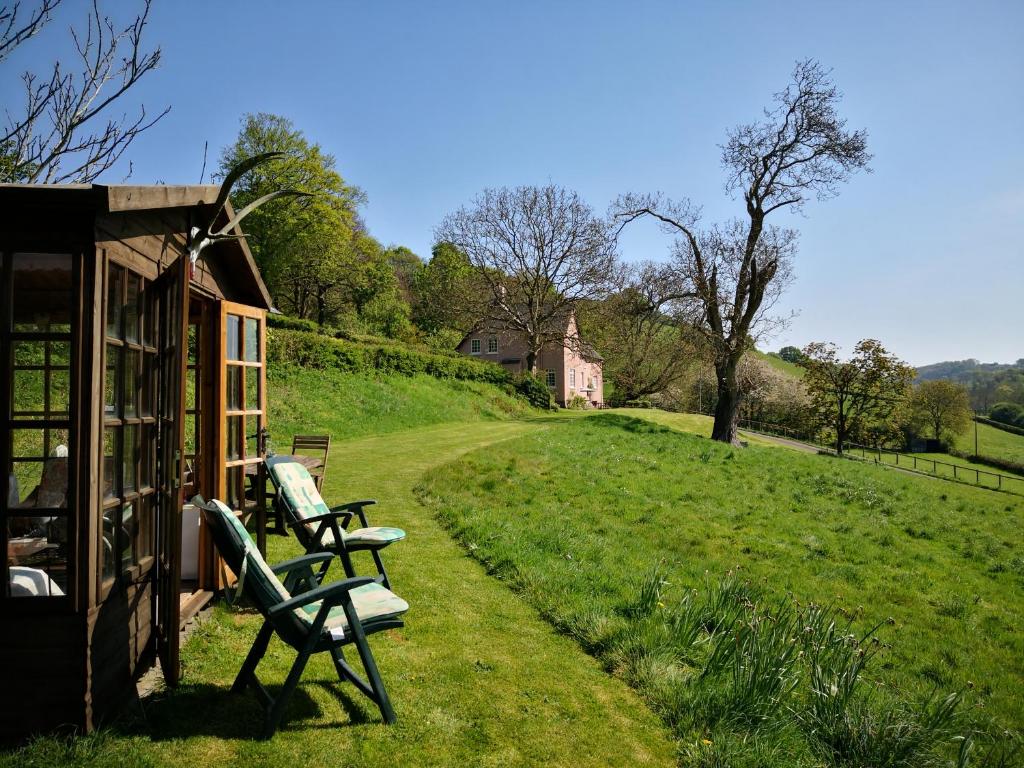In this outdoor daytime photographic scene, a detailed view showcases a one-story wooden cabin or shed with wooden frames and double doors located on the left side of the image. The structure's walls are largely composed of windows, giving it a greenhouse-like appearance, and there is an animal skull with long horns or antlers mounted over the top of the doors. These doors are open, revealing two cushioned wooden chairs positioned right outside.

A recently mowed walkway begins from in front of this smaller cabin and leads downhill towards a more substantial two-story brick house with gabled roofs, visible in the middle background. The cabin appears nestled in a grassy incline, surrounded by both trimmed and wild grass. A distinctive Y-shaped tree branches out almost directly in front of the cabin, adding to the picturesque countryside setting. 

The scene extends to showcase a blue, cloudless sky covering the top right corner, with rolling hills, and a variety of trees—some leafy and others bare—stretching across the middle distance. There is also a hint of a distant fence, blending harmoniously into this tranquil rural landscape.